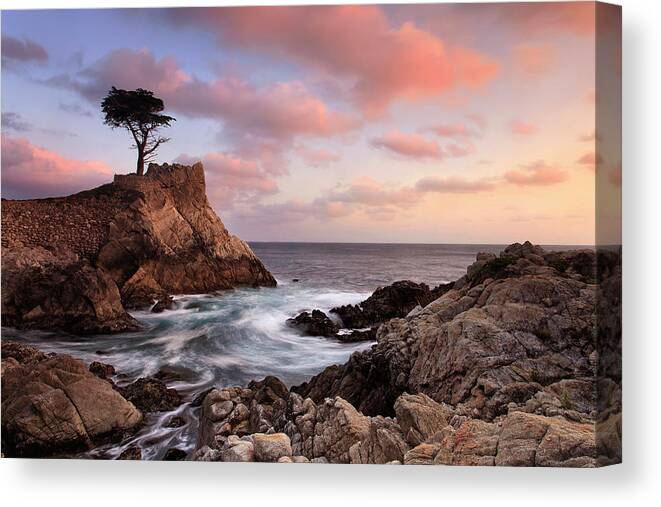The image depicts a serene coastal scene at sunset, characterized by craggy rock formations jutting into the water and a tranquil inlet. Taken from a perspective slightly to the right, the scene features a gradient sky transitioning from blue to orange and pink as the sun sets out of frame. A single, lone tree stands atop a cliff on the left, with sparse foliage only at its higher branches. The water gently flows between the rocky outcroppings, creating a harmonious and peaceful atmosphere. The entire composition is rendered on a wraparound canvas, giving it a realistic but artistic quality, with no human presence disrupting the natural beauty.